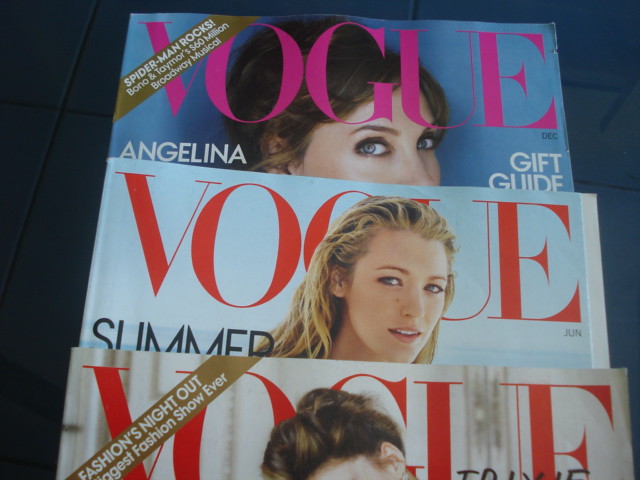The image is a color photograph in landscape orientation, featuring three overlapping issues of Vogue magazine, laid out on a dark navy blue table. The top magazine showcases the Vogue logo in bright pink with the title "Angelina" and various articles including "Gift Guide," "Spider-Man Rocks," and "60 Million Broadway Musical." The cover displays a woman with dark hair and blue eyes, reminiscent of Angelina Jolie, although her face is partially obscured. This is the December issue. The middle magazine, with the Vogue logo in red, features a blonde woman with wet hair, possibly suggesting a beach setting. This is the June issue. The bottom magazine, also with the red Vogue logo, is mostly cropped out, revealing only a woman's head with brown hair and headlines hinting at "Fashionist Night Out" and "Biggest fashion show ever."